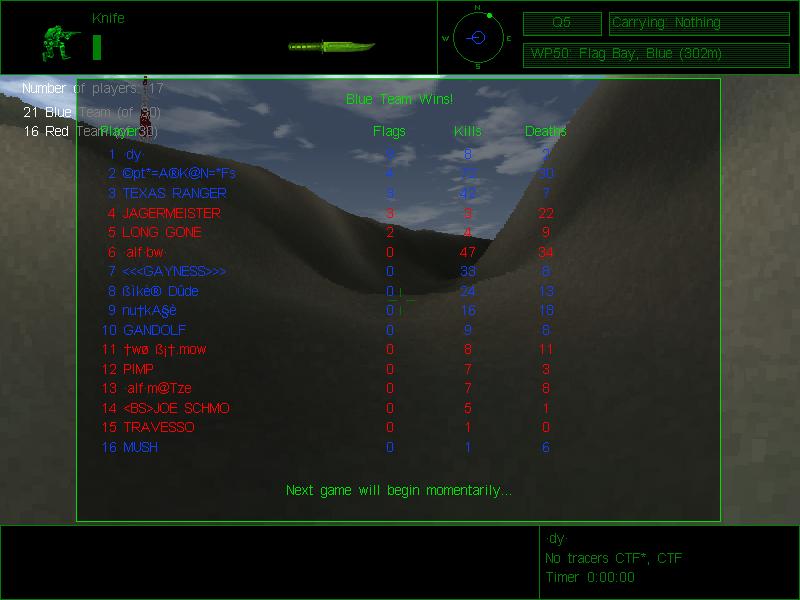This still image from a video game captures a tense moment in a desert landscape. In the background, sandy hills stretch across the horizon under a sky adorned with scattered white clouds, transitioning from light to dark blue tones. The sandy terrain appears in a darker gray hue, creating a stark contrast with the sky above. A prominent black band runs across the top of the screen, housing various game information.

On the far left, a small green character is shown crouching, poised with a rifle aimed to the right. Above him, the word "Knife" appears in green text. To the right center of the screen, an image of a dagger points to the right, indicating perhaps an item or an ability in the game.

The upper right corner features a compass, accompanied by text reading "Q5 carrying nothing" and "WP50 flag bay blue," providing context about the character's current status and objectives. In the center of the screen, game statistics are displayed, detailing the performance of the blue team with information on flags, kills, and deaths, along with a message stating, "Blue team wins." A notification at the bottom announces, "Next game will begin momentarily," indicating a brief interlude before the next match.